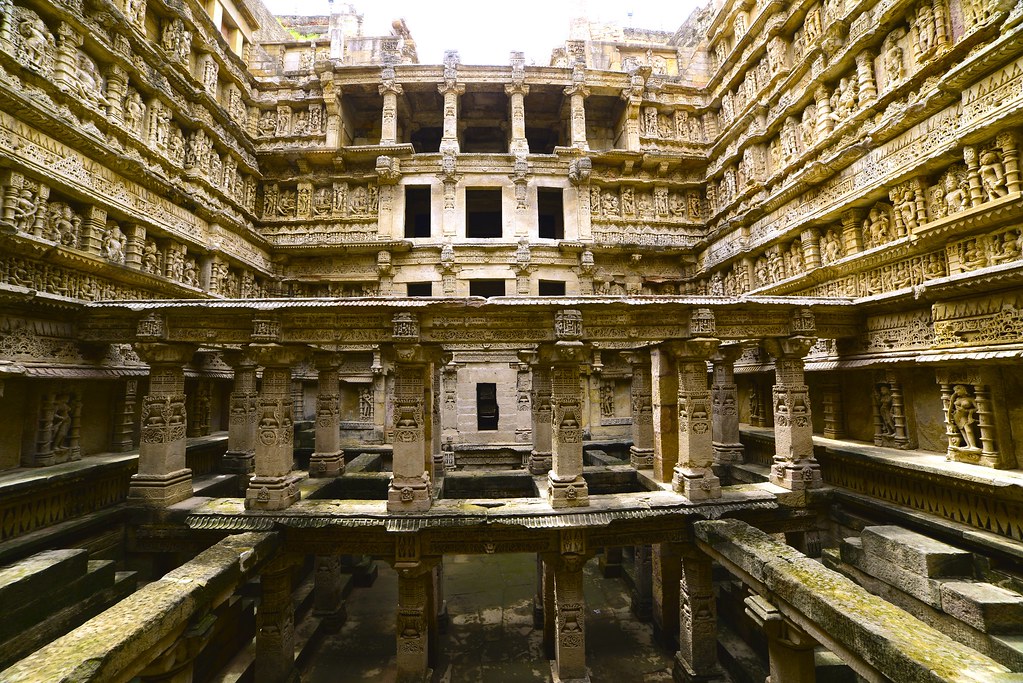This stunning, full-color photograph captures the intricate and awe-inspiring Queen’s Step Well, also known as the Rani Ki Vav, located in India. The scene is lit by natural daylight, highlighting the ornate, ancient architectural structure that appears to be crafted from light beige stone, giving it a gold-like appearance.

The image is a detailed view from the ground level, looking up into the central courtyard of this multi-storied marvel. The courtyard is framed by two walls on the right and left, which intersect with a back wall adorned with rows upon rows of finely carved columns and statues depicting humans, animals, and mythical creatures. These carvings extend across several floors, showcasing the ingenuity and craftsmanship of its creators. At the top floor of the back wall, the columns support a flat roof.

In the foreground, a small body of water—perhaps a river or pool—is visible, with a footpath or bridge crossing it. Concrete steps can be seen on the right side, suggesting access routes within the structure. There are no borders or background distractions, ensuring the focus remains on the step well’s architectural beauty and the elaborate carvings of its façade. The photograph, expertly utilizing natural light, brings out the vivid details and textures of this historical masterpiece, epitomizing representational realism.